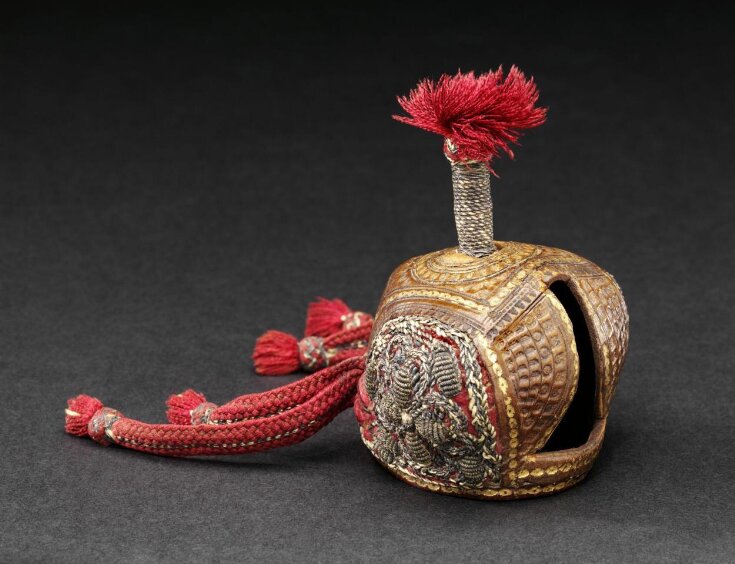The image depicts an intricately designed, golden helmet that resembles a medieval knight's hat or perhaps a regal falconry hood. The helmet is predominately gold with elaborate designs and features red accents. A distinctive feature is a small pole on top, adorned with a lens and a cluster of red string tassels, giving it an ornate and historic appearance. On one side of the helmet, a thick red rope culminates in a sweeping pattern of strands that further enhance the decorative detail. The background appears to be a plain gray carpet, providing a neutral contrast to the helmet's vivid colors and intricate craftsmanship. The overall aesthetic suggests a blend of historical and ceremonial influences, highlighted by the combination of gold with intricate red details.